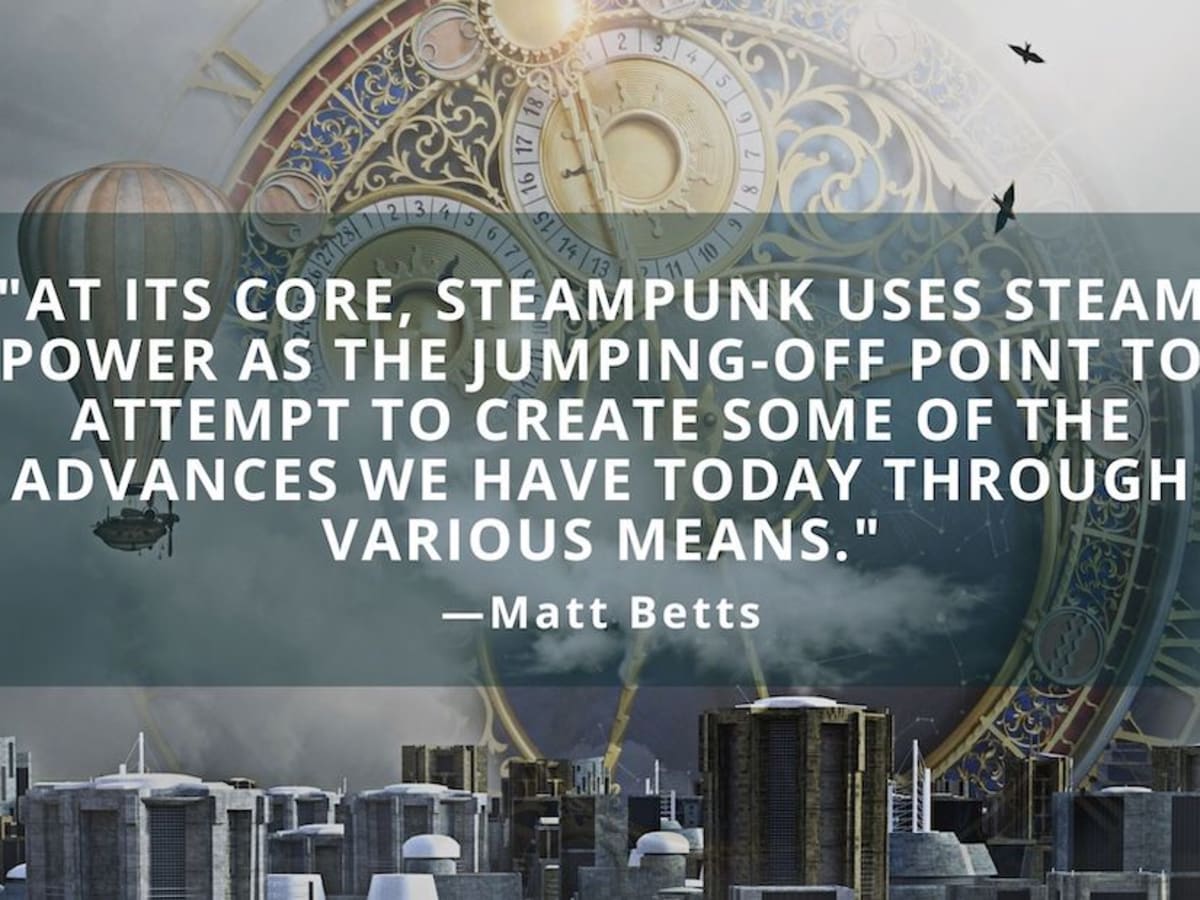The image features a cityscape at the bottom with smaller buildings colored in silver, white, and brown, some of which have antennae or spikes on their rooftops. Overlaying this cityscape is a central piece of text by Matt Betts that reads, "At its core, Steampunk uses steam power as the jumping off point to attempt to create some of the advances we have today through various means." The text is in white and prominently printed in the middle of the screen. Behind this quote lies an elaborate astrological clock adorned in gold, blue, maroon, and white hues. To the left of the clock, a unique blimp with a ship attached underneath adds to the scene's historical yet futuristic aesthetic. Birds are seen flying in the top right corner, enhancing the dynamic feel of the image. The setting blends a 1890s vibe with futuristic elements, highlighted in muted and vibrant colors like yellow, blue, maroon, and red.